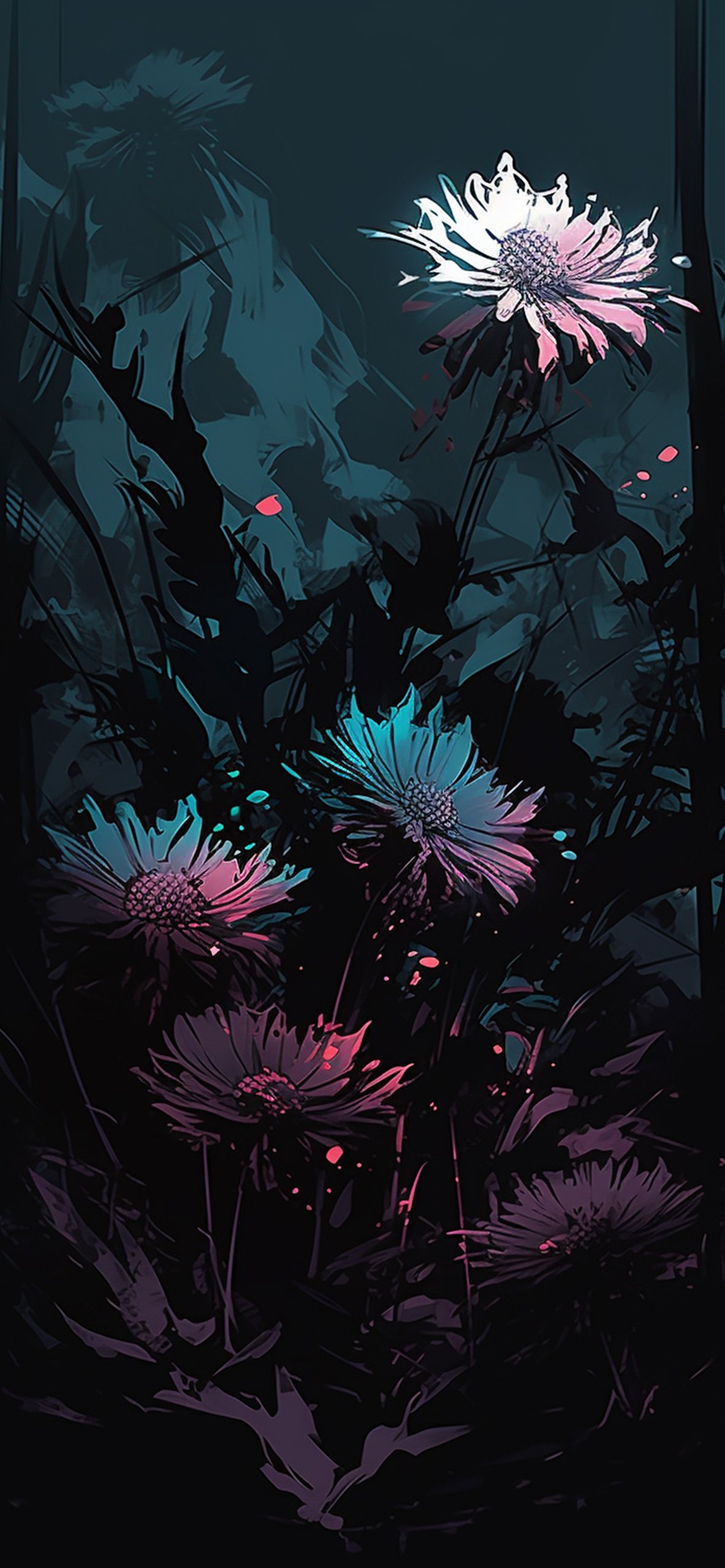The artistic piece is a vertically rectangular, multi-color print without a set border or background, resembling a dark digital illustration. The main focus is an artist's abstract interpretation of daisies interspersed with silhouettes of ferns or vines. The background shifts from a lighter blue on the upper left side to dark grey, dark blue, and eventually, pure black at the bottom. In the upper right-hand corner, there's a white daisy-like flower tinged with pink, illuminated as though by a spotlight. Below it, successive flowers display hues transitioning from light blue and pink to darker purples and reds as they descend. The lowest flower, situated towards the bottom left, is a deep purplish-red. Scattered throughout the painting are sporadic dots of red and blue, adding a touch of whimsy to the otherwise dark and moody composition. The flowers and plants become darker and more indistinct towards the bottom, where the background ultimately dissolves into blackness.